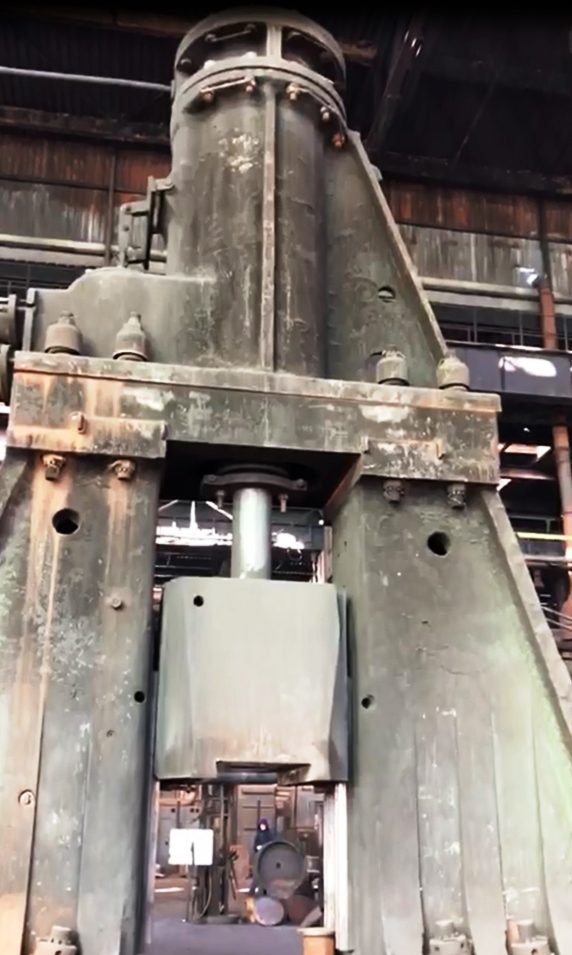This photograph captures a towering, industrial hydraulic press with a massive, bulky steel frame, prominently featuring immense bolts on the sides and a colossal pipe descending from the top. This hydraulic pipe merges into a large steel cylinder centrally situated, which extends to a thick square steel block at the base of the machine. The machinery is heavily weathered, adorned with patina and extensive rust, giving it a timeworn appearance. The image, taken in portrait mode, reveals a factory setting, with metal catwalks in the background and additional machinery and hosing visible through the open space beneath the steel block. The entire structure is gray and metallic, with streaks of copper patina marking its surface, emphasizing its age and industrial use. The press, standing imposingly within a cavernous warehouse-like environment, appears capable of accommodating people walking under its elevated components.